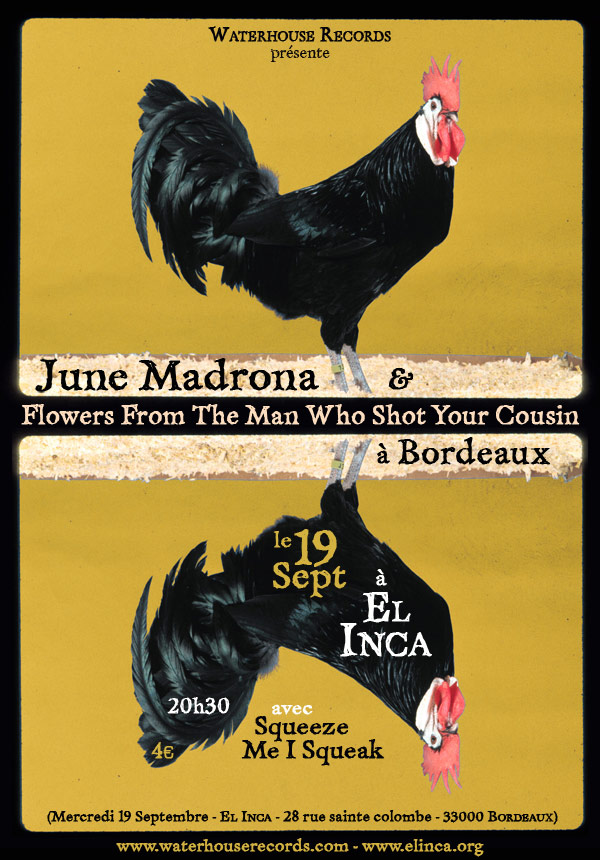The promotional poster, illustrated with bold and contrasting colors, features a mustard background framed with a black border. The top half prominently contains the text "Waterhouse Records, Présente" above a striking line-art depiction of a black rooster with a red comb. Positioned to the left of the rooster, the names "June Madrona and Ah Bordeaux" are displayed. Below this, on a horizontal black band demarcated by beige borders, reads the intriguing phrase "Flowers from the Man Who Shot Your Cousin."

The bottom half mirrors the top with an upside-down reflection of the rooster, detailed with mustard-colored text "Lee 19 Sept" and white text "A. L. Inca" overlaying the image. To the left of the inverted rooster, the time "20 H. 30" is specified. Beneath the rooster, against the mustard background, further text proclaims "Avec Squeeze Me I Squeak." Anchoring the poster at the very bottom are the URLs "www.waterhouserecords.com" and "www.elenia.org." The combined elements of imagery and typography deliver a visually compelling announcement, replete with details that entice and inform the audience.